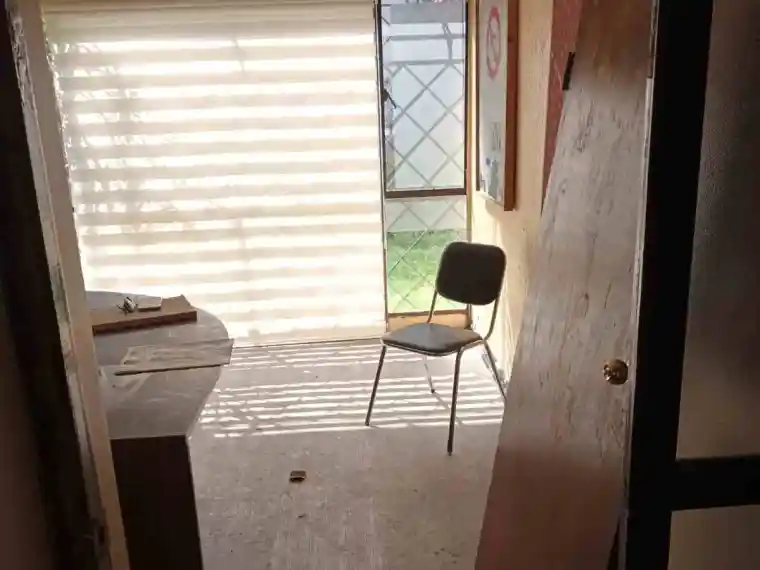The image captures a view through a doorway into a small, abandoned office bathed in the fading light of the setting sun. The door, a wooden one that is now off its hinges, leans haplessly against the frame. The room is notably sparse, dominated by brown, gray, and orange hues, lending it a dingy and forlorn appearance. To the right of the doorway, a solitary 80s-style chair sits askew off-center, adding to the sense of desertion. The floor is bare, devoid of any carpet or linoleum, revealing its plain, unadorned surface. A wood desk stands against one wall, with a book and some paperwork left abandoned on top of it. Above the desk hangs a single, unidentifiable poster or framed artwork. Blinds or shades cover the window on the sidewall, through which the late evening sun casts long, somber shadows into the room. Adjacent to the window is a small sidelighted window that possibly opens with a latch. The ethereal, mysterious ambiance provokes curiosity about the past events that led to the office's current state of disuse.